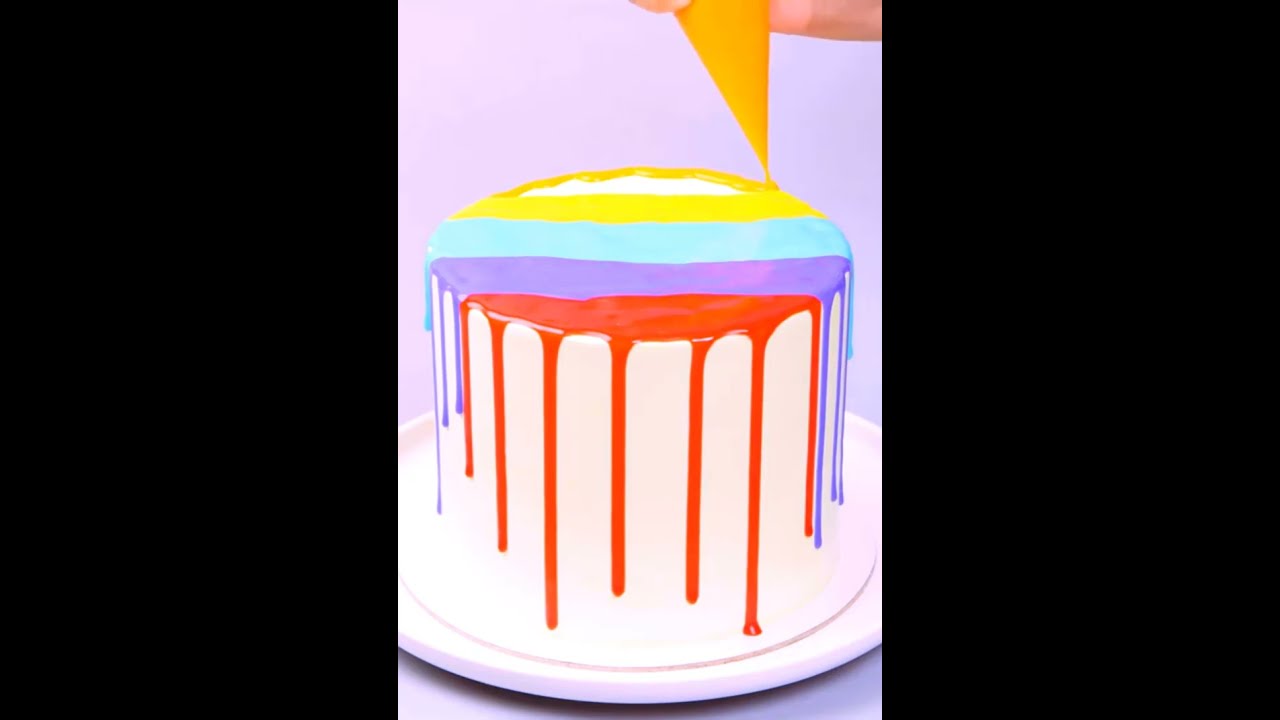This image depicts a tall, rounded white cake on a white plate, set against a lilac background. The cake appears to be in the midst of being decorated, with a hand holding a piping bag filled with orange icing at the top right of the picture. The colorful icing, which includes red, purple, blue, and yellow, artistically drips down the sides of the cake, creating a vibrant, cheerful effect. The orange icing from the piping bag is actively being applied, adding to the array of colors. The cake has a tiered look, suggesting multiple levels. The image has a distinctive style, possibly a photograph taken with a cell phone or a graphic design, indicated by the wide black borders on the left and right, partially obscuring the cake and plate. The cheerful, colorful scene evokes an almost celebratory or pride-like vibe.